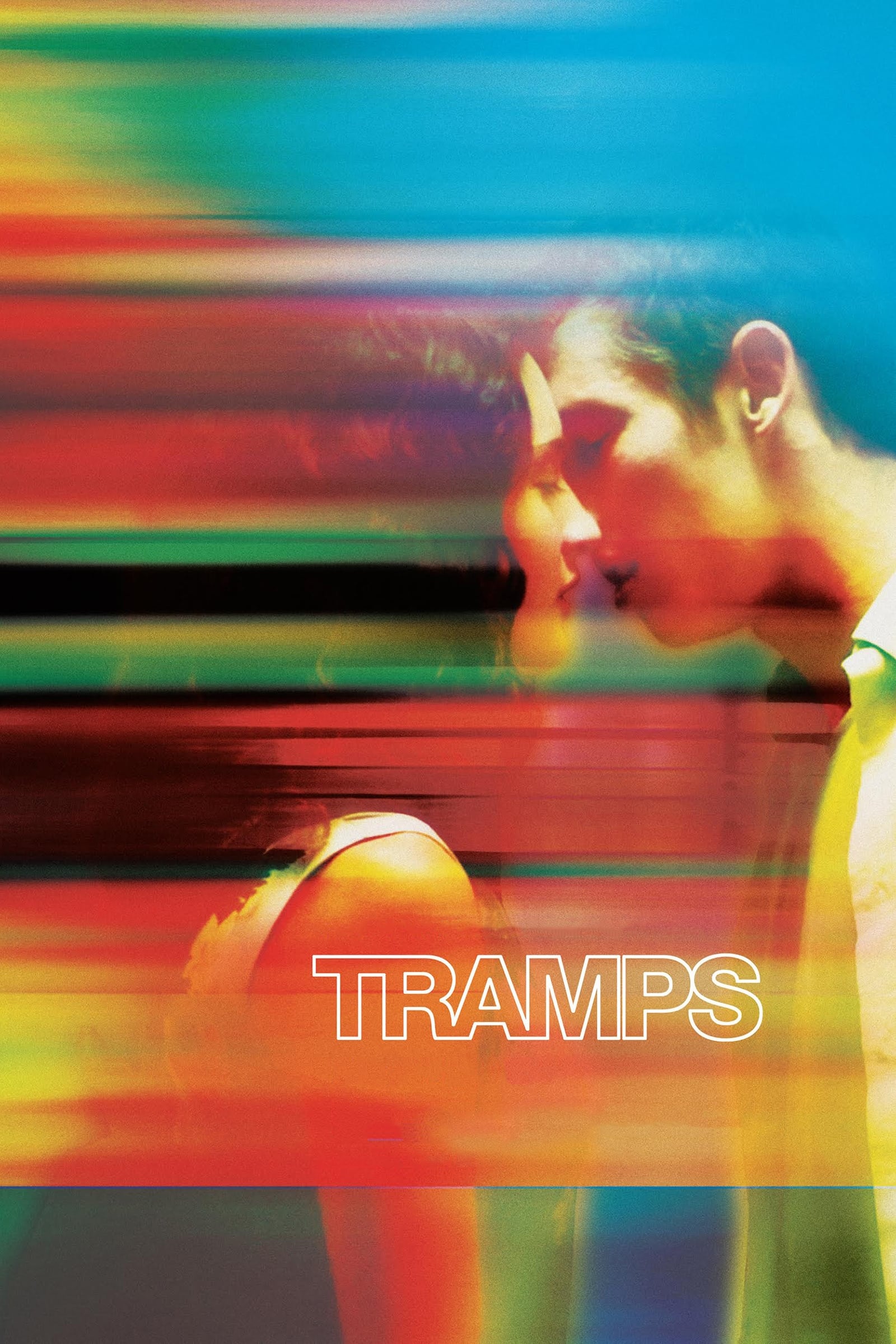A vibrant and colorful image features a man and a woman positioned close together in the center, as if about to kiss. The background is a blend of horizontal stripes with a gradient from blue at the top, transitioning to pink in the center, and solid shades of purple, red, and green towards the bottom. The colors are mixed with overtones of blues, reds, pinks, yellows, and greens, giving it a rainbow-like, blurred effect.

The woman, positioned on the left, has long, wavy hair that reaches past her shoulders. Her eyes are closed, and she faces the man, wearing a sleeveless top that reveals her right arm. She has a light complexion. The man, slightly taller and standing on the right, has short black hair and a similar complexion. He is facing the woman with eyes closed, wearing a collar shirt that appears yellow or white, possibly altered by the colorful overlay.

At the lower mid-right part of the image, the word "TRAMPS" appears in all caps with a white outline, suggesting that this could be a poster or an advertisement, possibly for a movie. The entire scene is slightly faded, enhancing the effect of closeness and intimacy between the two figures amidst the colorful, blended backdrop.